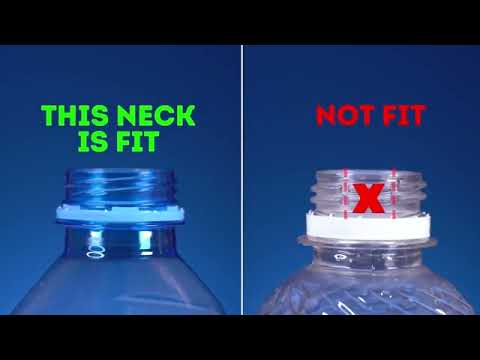The image is a comparative demonstration of two plastic water bottles placed side-by-side against a dark blue gradient background. The bottle on the left is tinted blue-green and features a green band around its neck, which fits the bottle’s screw threads. Above it, in lime green text, it says "This neck is fit." There is a white reflection present on part of this bottle. The bottle on the right is clear with a white plastic band around its neck, which does not fit properly. Above this bottle, in red text, it says "Not Fit," and a bold red X, flanked by two vertical dotted lines, marks the neck to indicate the mismatch. Both bottles have the same bluish-gray background.